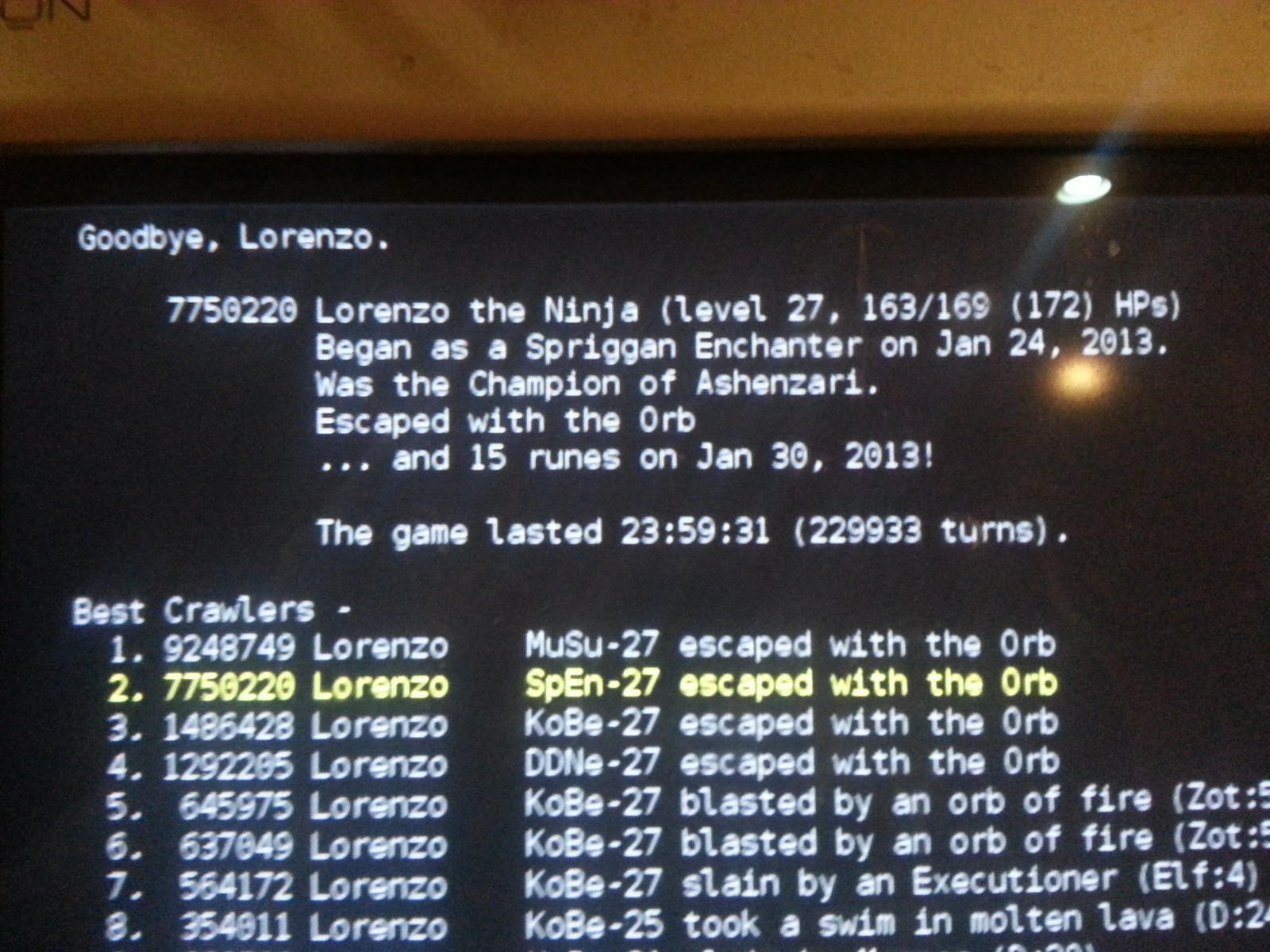The image features a close-up view of a screen, possibly from a computer or a projection. It is clearly indoors in a dimly lit room, with a visible portion of the ceiling and a single light source illuminating the scene from the top right. The screen occupies the center of the photo, displaying text that indicates it is from a text-based game. The screen's background is black, and the majority of the text is white, except for one standout line in yellow, indicating the player's ranking.

The text details the accomplishments of a player named Lorenzo, dubbed "Lorenzo the Ninja," who reached level 27 as a Spriggan Enchanter. Lorenzo began this character on January 24th, 2013, and completed a noteworthy feat by escaping with the orb and 15 runes on January 30th, 2013, after a game that lasted 24 hours and accrued 229,933 turns. This resulted in Lorenzo achieving the second place on the leaderboard. The colors in the image consist of black, white, yellow, gray, and brown, contributing to the overall muted, focused ambiance of the setting.